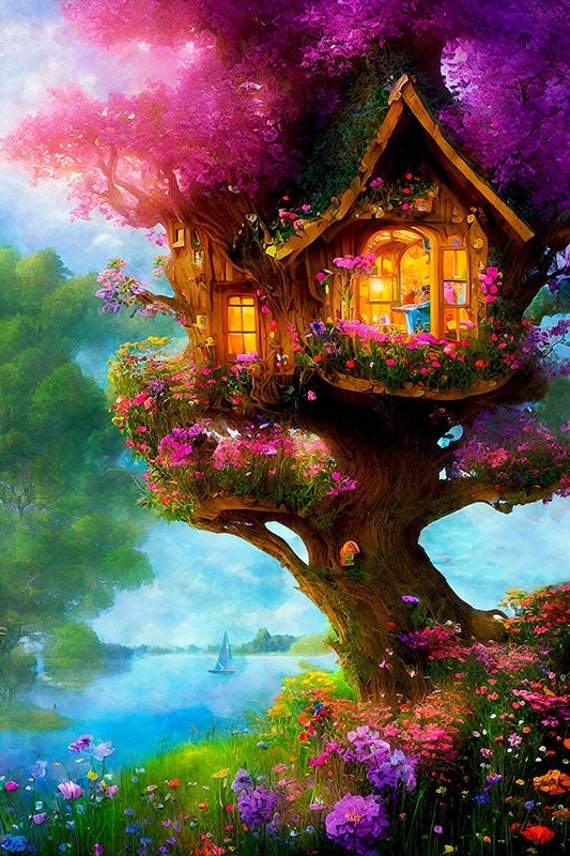The image depicts a whimsical, elaborately constructed treehouse nestled within a vibrant, fantastical tree. The tree itself is adorned with fluorescent pink and purple leaves, lending a distinctly cartoony and surreal feel to the scene. The treehouse stands out with its A-frame roof, partially overgrown with greenery, and features two windows—one open, with shuttered panels, and one closed. Inside the treehouse, a softly glowing yellow light illuminates the interior, and through the open window or door, a figure—possibly a child in a blue outfit—is faintly visible.

Surrounding the treehouse, a riot of colorful flowers flourishes, with hues ranging from deep reds and purples to bright pinks and whites. These blooms cascade down the branches of the tree and gather densely around the base, creating an enchanting floral display. The trunk of the tree features a tiny doorway, painted in yellow and green, though its details are somewhat obscured. 

The background showcases a tranquil, hand-painted sky, with fluffy white clouds against a serene blue. A stream or river flows from the bottom right of the image toward the middle horizon, where a sailboat floats gracefully. To the right of the scene is a partially visible plain green tree, adding a touch of contrast to the fantastical setting.

This ethereal, computer-generated or watercolor-enhanced scenery, with its vivid and fluorescent palette, exudes a dreamlike, fantasy quality, making it a captivating portrayal of a magical treehouse retreat.